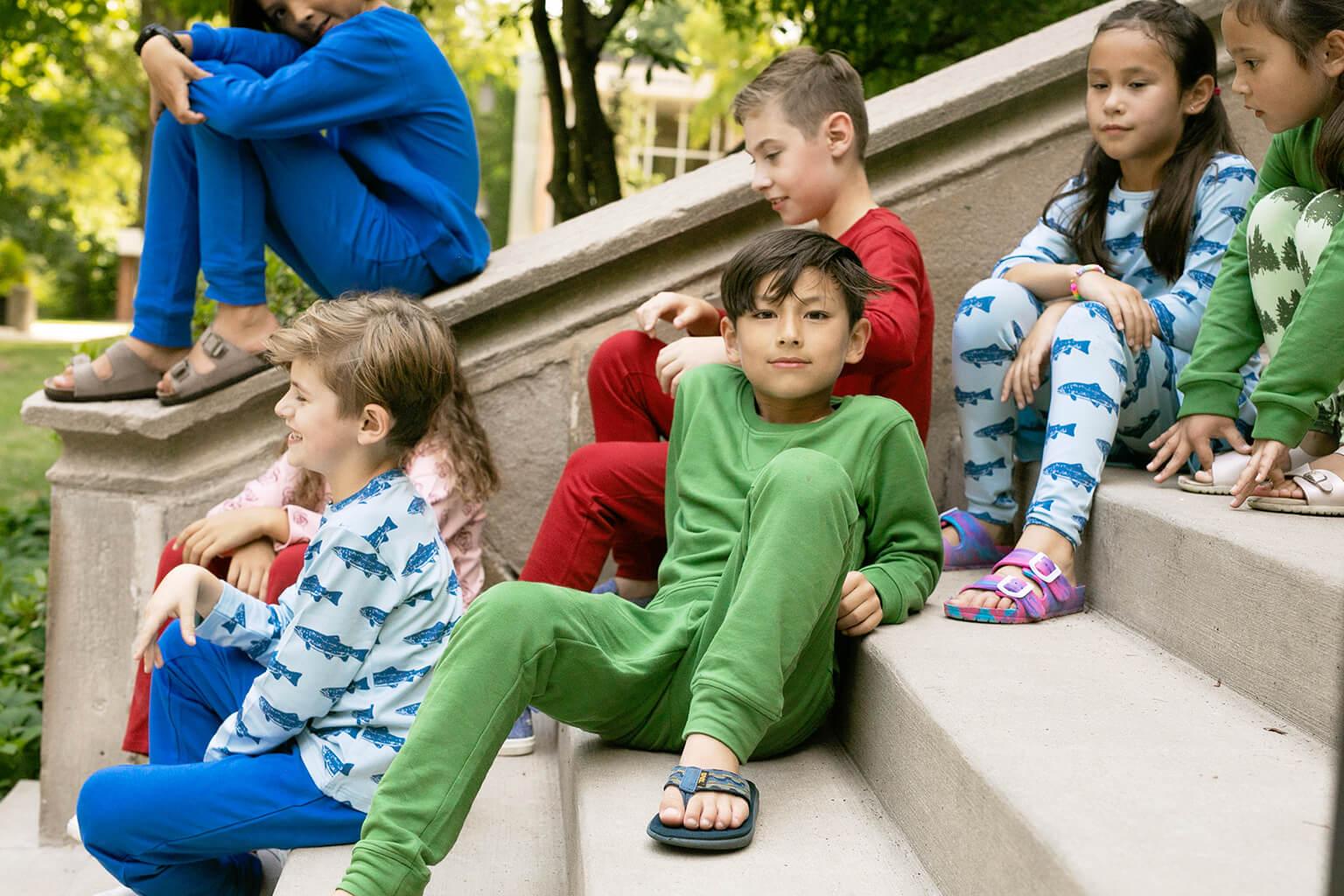The image depicts a group of children casually gathered on a set of concrete stairs outdoors during the daytime. The central figure is a boy with a light tan, wearing green, long-sleeved pajamas that resemble a onesie, paired with sandals and no socks. He has straight brown hair, brown eyes, and is smiling directly at the camera, creating a direct connection with the viewer. Surrounding him are a mix of boys and girls, all also dressed in various styles of pajamas. Two girls sit slightly above him on the steps, while another child is positioned behind and beside him. In front of the central boy are two more kids, and one additional child perches on the railing of the stoop. The scene exudes a sense of camaraderie and childhood innocence, accentuated by the casual attire and outdoor setting under broad daylight.